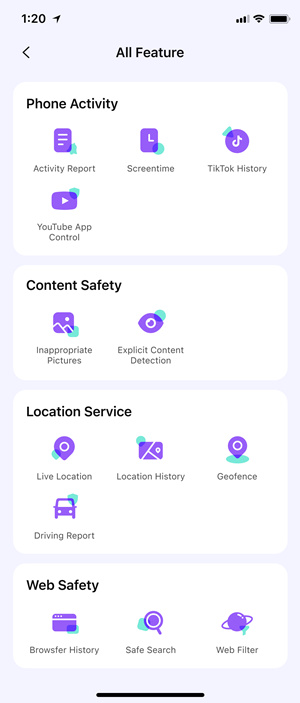The image shows a detailed phone interface with a light blue background and black text. At the top, the number "120" is displayed with an arrow pointing up and to the right, alongside another arrow pointing to the left. Below, the interface is divided into various sections.

The first section is titled "All Features" and contains a large white box labeled "Phone Activity." Inside this box, there are several blue icons:
1. A blue sheet of paper with a blue circle labeled "Activity Report."
2. A blue clock with a similar circle beneath it labeled "Screen Time."
3. A blue square with a blue-green arrow labeled "TikTok History."
4. Another blue square with a white arrow pointing to the right labeled "YouTube App Control."

The next section is titled "Content Safety" with another white box containing:
1. An icon resembling blue waves with a white head, and a green spot labeled "Inappropriate Pictures."
2. An icon of a blue eye with a green spot labeled "Explicit Content Detection."

Another large white box labeled "Location Service" follows, containing:
1. An icon shaped like a rounded blue thing with a tipped edge and a green spot labeled "Live Location."
2. A blue icon with a green spot labeled "Location History."
3. An icon shaped like a pointed, round thing with a green circle beneath it labeled "Geofence."
4. A blue car with a green circle labeled "Driving Report."

The final white box is labeled "Web Safety" and includes:
1. A blue icon with a green circle labeled "Browser History."
2. A blue icon with a green square labeled "Safe Search."
3. An icon of a blue Earth with a green spot labeled "Web Filter."

The entire interface appears streamlined, with blue and green icons providing visually distinct functionalities related to phone activity, content safety, location services, and web safety.